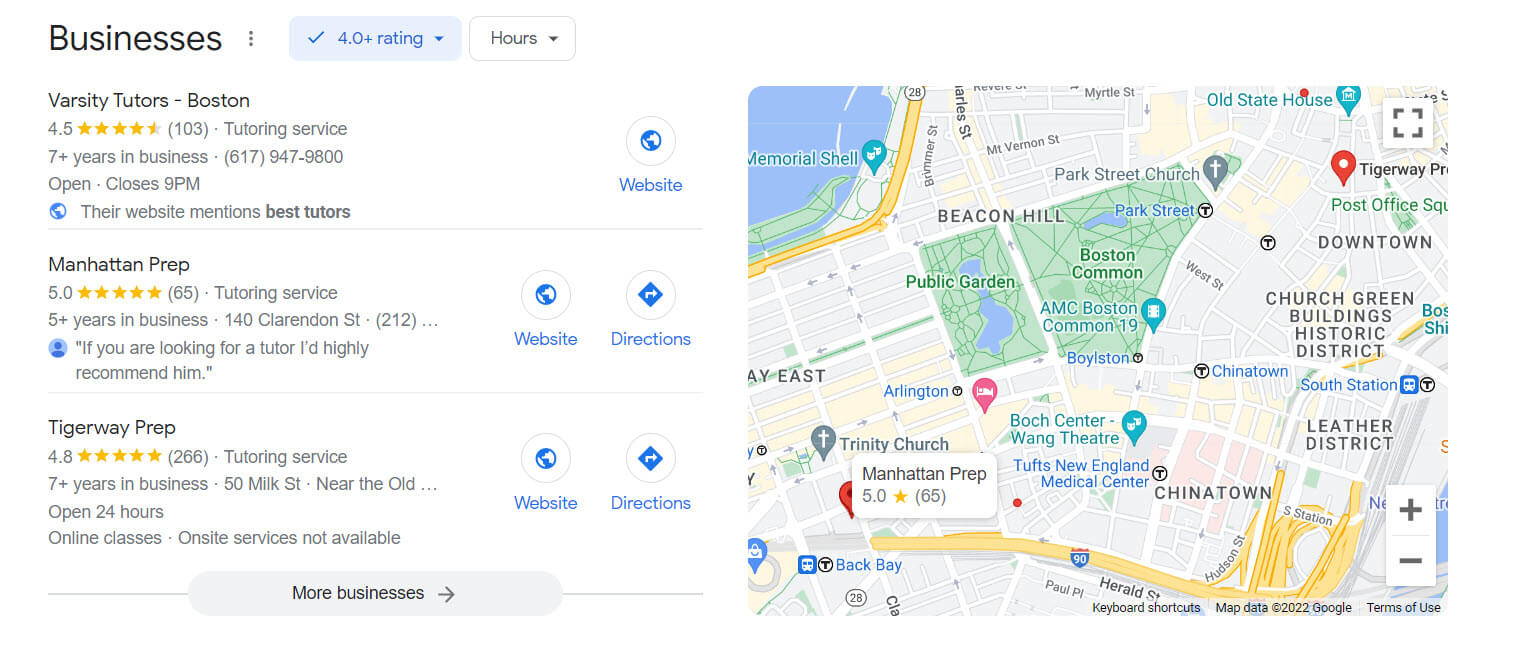A detailed screenshot captures a comparison of three educational services in Boston, with their ratings and reviews prominently displayed. Varsity Tutors Boston boasts a rating of 4.5 from 103 reviews, while Manhattan Prep shines with a perfect 5.0 from 65 reviews. Tiger Way Prep has an impressive rating of 4.8 from 266 reviews. To the right of Varsity Tutors Boston is a clickable "Website" button, while Manhattan Prep and Tiger Way Prep each have both "Website" and "Directions" buttons. Below these details, a gray rectangle suggests more options with an arrow indicating more businesses available for viewing. On the right side of the screenshot, a map displays the locations of Manhattan Prep and Tiger Way Prep, but Varsity Tutors Boston is not visible on the map.